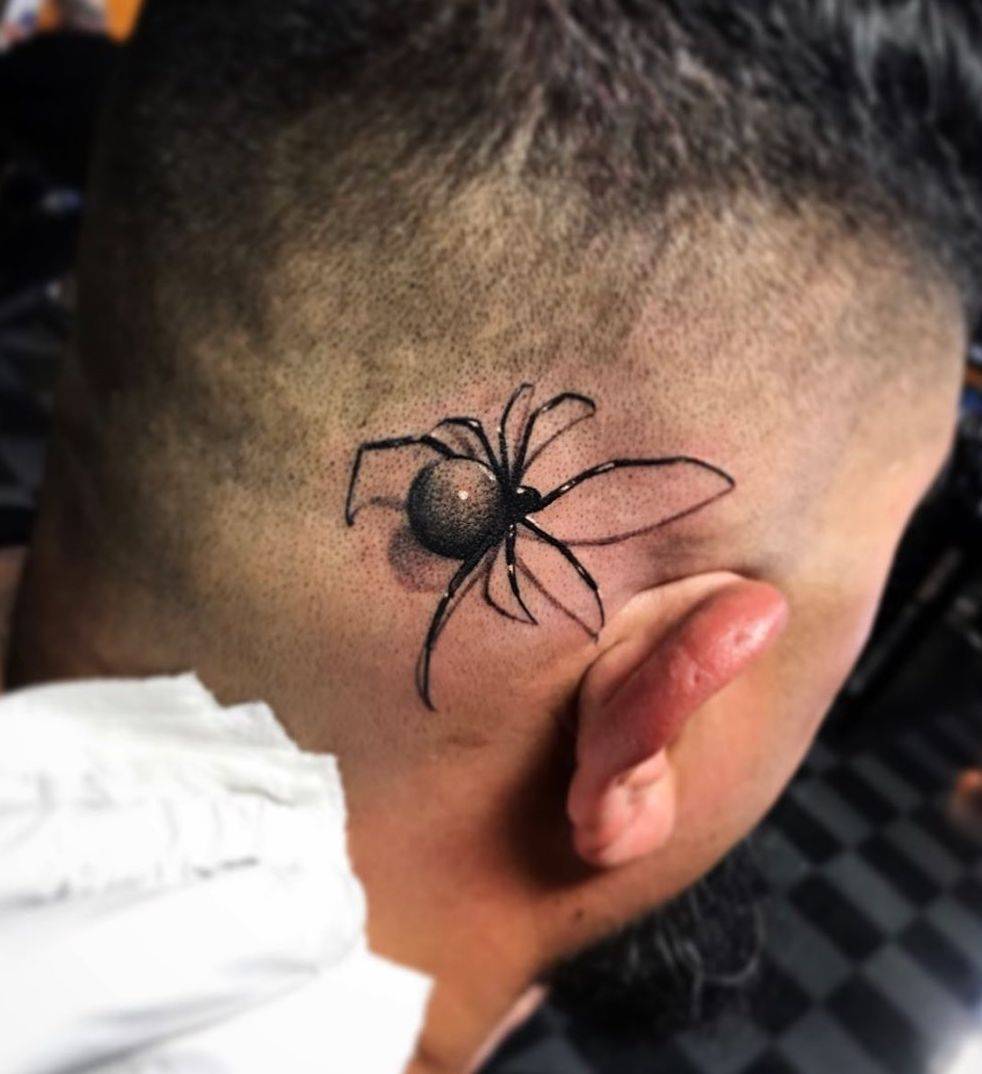The image shows the back right portion of a white male's head, with his hair closely cropped into an almost mohawk style, leaving the area behind his right ear shaved to make room for a large, fresh tattoo of a black spider. The spider, resembling a black widow but without the characteristic red marking, spans from behind the right ear to nearly the back of the head, and is facing toward the forehead. The surrounding skin appears red and irritated, indicating the tattoo is recent. Visible in the lower left-hand corner is a white towel used to wipe away excess ink. The overall scene suggests the tattoo is being applied in the moment, with the man tilting his head forward and away from the camera, revealing a dark shadow on the lower right corner of the image, possibly from the man's hair or the environment.